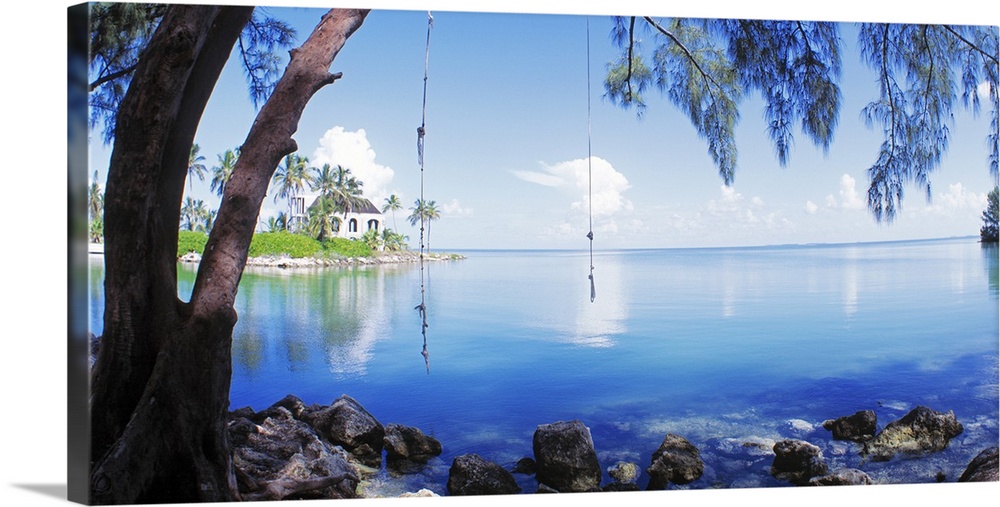The image depicts a vivid, tropical shoreline scene, meticulously printed on canvas and wrapped around a solid, inch-thick frame, giving it a pronounced presence on the wall. In the foreground, a desolate tree stands prominently, its branches and leaves stretching out and partially obscured by fishing line and tackle entangled from unfortunate fishermen. Surrounding the tree are rocks that peek out from the edge of a calm, blue lagoon. The water extends toward a distant promontory on the left, where a thatched roof hut or house is nestled among lush palm trees and vibrant greenery, creating the impression of a serene tropical island retreat. This building, possibly a small chapel, is complemented by a rock wall or jetty that connects it to the tranquil, azure ocean. Above, the sky is a brilliant blue, dotted with drifting white clouds that mirror on the water’s surface. The overall ambiance is one of peaceful isolation, enhanced by the detailed representation of the diverse elements, from the fishing debris on the tree to the idyllic shoreline, capturing the essence of a remote island paradise.